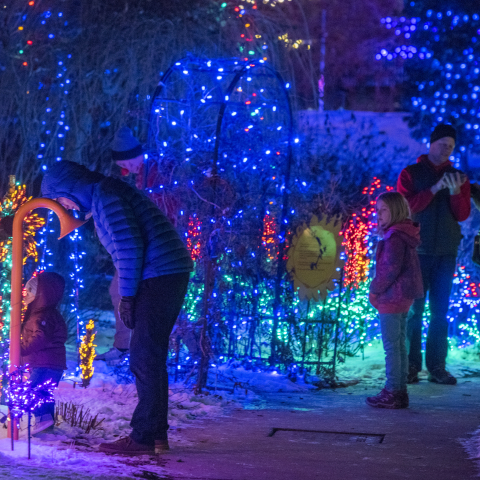The photograph, taken outdoors at nighttime, depicts a family of four—two adults and two children—standing in a snow-covered garden path area adorned with Christmas lights. Predominantly blue lights illuminate the scene, interspersed with smaller, brilliant yellows and golds. The right side of the image features a Caucasian man engrossed in his phone. To his left, a young blonde girl, also Caucasian, watches intently. An adult, possibly the mother, wearing a blue jacket, bends over at the waist, leaning her head on a metal pole that emerges from the ground. Next to her, a young boy is seen with his tongue stuck to the same pole. The surrounding scene includes archways and foliage, and a distinct metal gate, alongside a yellow sun ornament decorated with Christmas lights, completing the festive winter tableau.